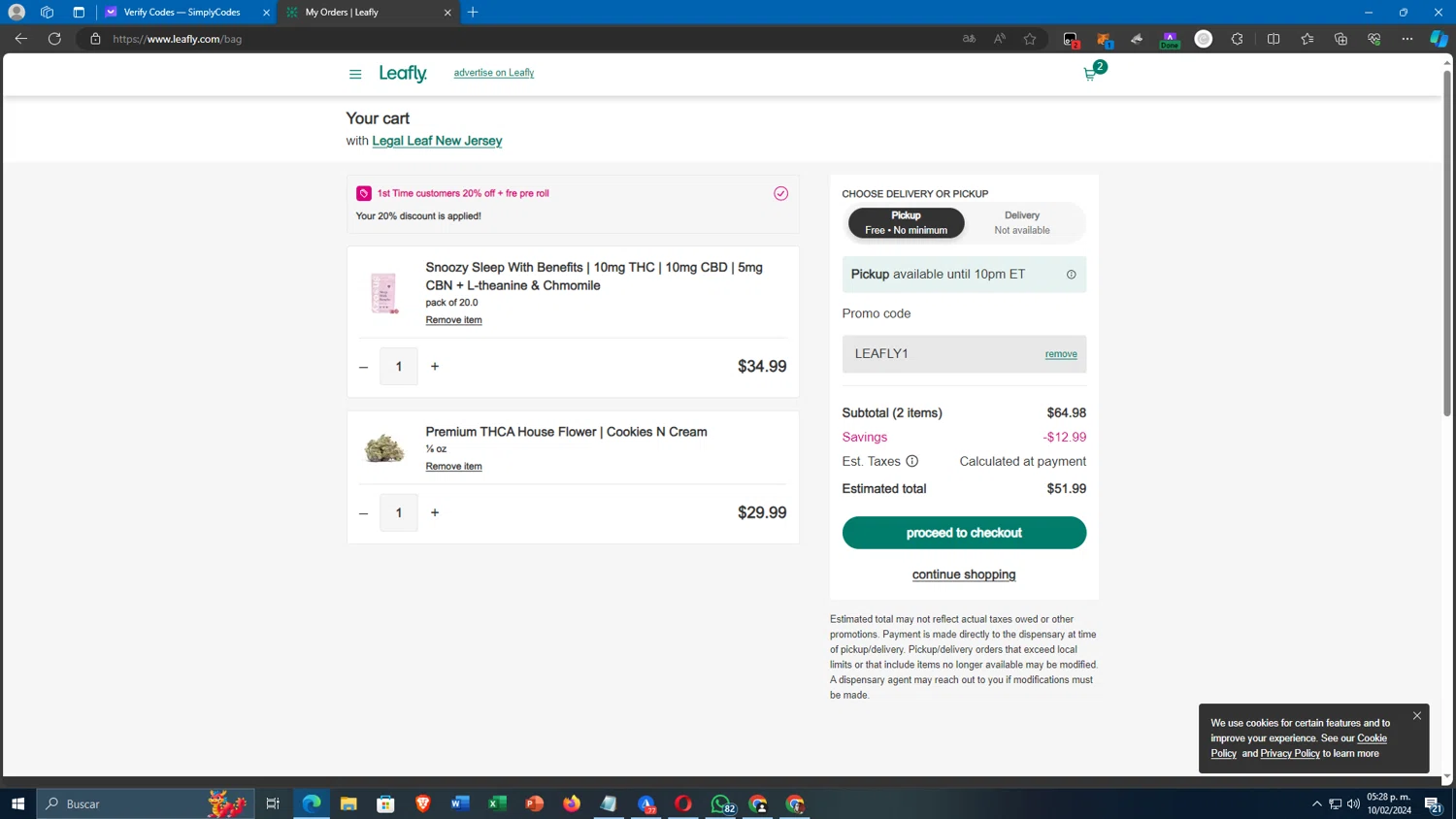A screenshot captured from an open Internet Explorer browser window, displaying two tabs at the top, though their small size makes the text difficult to discern. The active tab is labeled "My Orders, Weefly" and is highlighted in gray. Below the tabs, the browser's address bar shows the URL: "https://www.weefly.com/". 

The main content of the webpage features a gray header bar followed by a white navigation bar containing the site name "Weefly" and a shopping cart icon with a badge indicating 2 items. Directly beneath this, another white bar displays "Your Cart" alongside the text "Legal Leaf New Jersey". 

The cart items are listed in distinct white rectangles. The first item is "Snoozy Sleep with Benefits," which includes 10mg of THC, 10mg of CBD, and 5mg of CBN, complemented by L-theanine and chamomile, priced at $34.99.